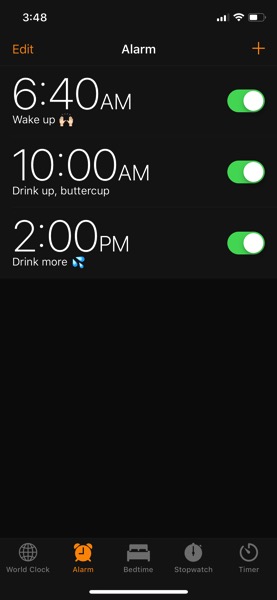The image displays a digital interface against a black background. In the top left corner, the time "3:48" is shown, while the top right corner indicates "3 out of 4 signal bars," a "full WiFi signal," and a "half-full battery" icon alongside an "alarm" label. An orange "Edit" hyperlink and an orange plus sign (+) appear below these indicators. 

Centrally, the large text "6:40 AM" is prominently displayed, with a smaller "Wake Up" label underneath. To the right of this, a green toggle switch indicates that the alarm is activated. 

Subsequently, the text "10:00 AM - Drink up buttercup" is shown, similarly accompanied by a green toggle switch on the right. Further down, "2:00 PM - Drink more" is listed with another green toggle switch activated.

Towards the bottom of the interface, a black rectangular section transitions into a grey area. This grey area contains navigation options: "World Clock," "Alarm," "Bedtime," "Stopwatch," and "Timer," with the "Alarm" option highlighted in orange, indicating that it is currently selected.